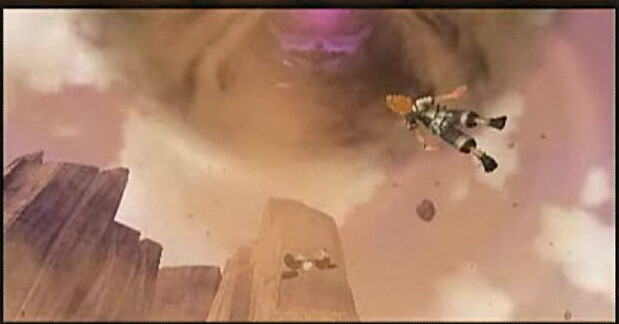In this detailed screenshot from what seems to be a contemporary video game, we observe a vibrant and immersive landscape, characterized by the presence of several rugged mountains and steep cliffs predominantly colored in shades of brown and gray. The sky above is similarly hued, presenting a somber atmosphere. Central to the scene is a striking, otherworldly phenomenon—a large, swirling vortex or portal with an intense purple core opening up amidst the cloudy sky. Adding to the dynamic nature of the image, we notice a slightly blurred figure resembling a humanoid character, seemingly airborne, either flying towards the vortex or being drawn into its gravitational pull. The overall high-quality graphics of the image, typical of modern video games, contribute to the depth and realism, while the scene itself is devoid of any textual elements, allowing the viewer to focus entirely on the dramatic visual portrayal.